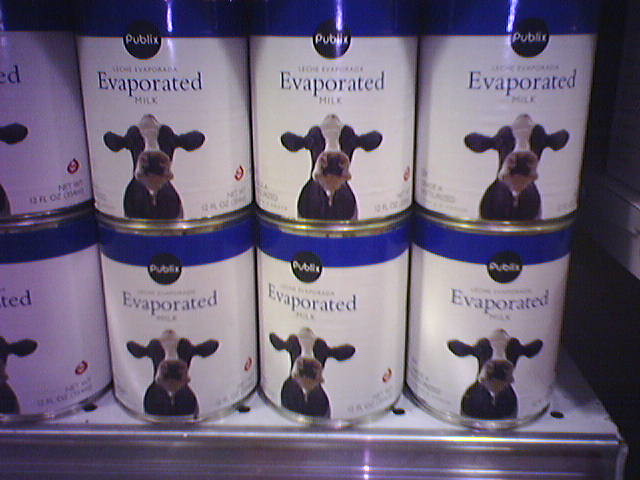The image captures a well-organized section of a refrigerated grocery store aisle. The focal point is a neatly arranged display of evaporated milk cans, stacked precisely on a white shelving unit. The shelf itself is slightly elevated, with a shimmering, metallic base visible at the very bottom, adding a clean, modern aesthetic to the store environment.

Each can of evaporated milk is adorned with a beige label featuring an image of a black-and-white cow's face and front body, almost resembling a selfie. The cow's gaze is directed straight ahead, creating an engaging and somewhat whimsical visual element. The cans are predominantly white with blue lids, adding a pop of color to the neutral label. At the top of each label, a black circle prominently displays the word "Publix" in white, confirming the brand identity associated with the grocery store.

The display consists of two rows of cans, with four cans on the bottom row and four on the top row. However, the arrangement is slightly asymmetrical as the leftmost can is partially cut off, revealing a total of six fully visible cans. This meticulous yet slightly imperfect layout highlights the store's effort to maintain a visually appealing and inviting atmosphere for shoppers.